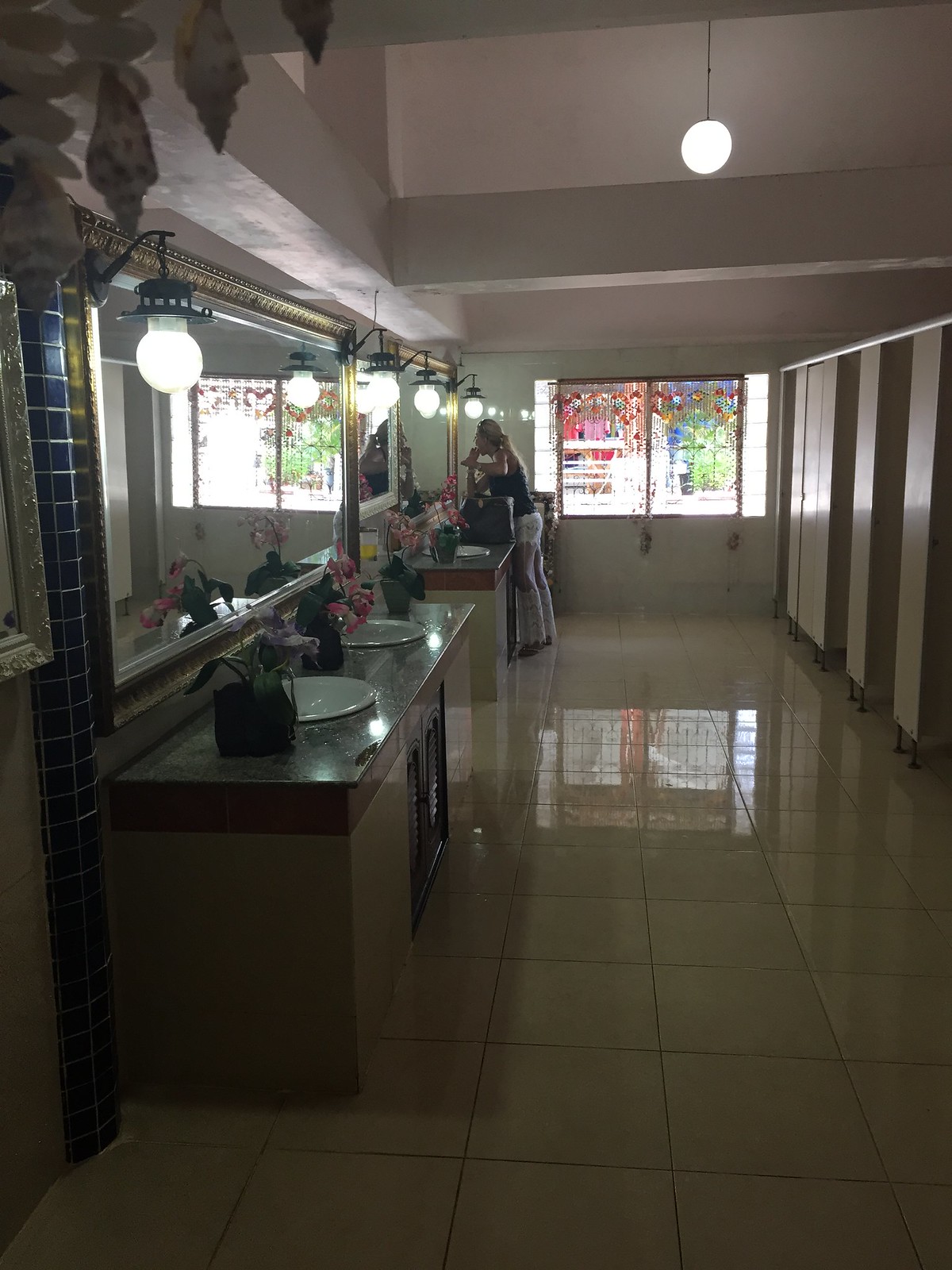This photograph is taken inside a public restroom, showcasing a well-lit, upscale interior. On the right side of the image, there are at least six beige-colored stalls with slightly elevated bases anchored into the floor, with the next to last stall being closed. The left side of the restroom features a series of countertops with a dark marble finish and ornamental gold-bordered mirrors above them. There are four porcelain white sinks arranged in pairs on the counters, each adorned with flower arrangements featuring colorful blooms in dark vases.

A variety of lighting fixtures illuminate the space, including round bulb lights hanging from the ceiling and additional decorative sconces on either side of the mirrors. The floor is covered in large, shiny, white tiles that reflect light from a large window at the back of the room. The window, adorned with beaded curtains, provides a glimpse of trees and possibly a shop outside.

A woman, who has blonde hair tied in a ponytail, is standing towards the back of the restroom. She is dressed in jeans, black sneakers, and a black tank top, seemingly applying makeup with her bag placed on the counter. The restroom exudes a clean and sophisticated ambiance, with its combination of high-end materials, decorative elements, and thoughtful layout.